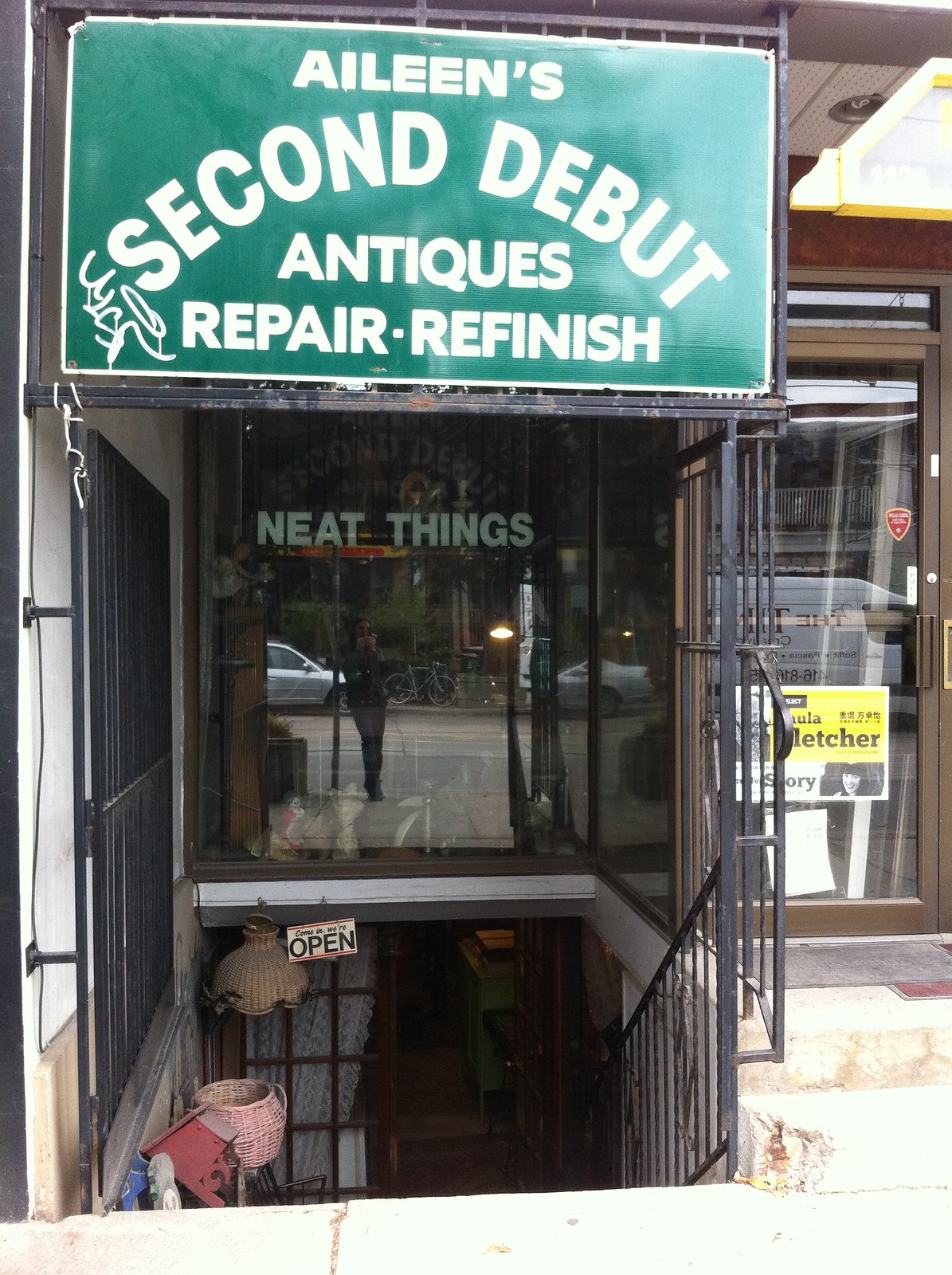The photograph captures an outdoor city scene featuring the storefront of "Eileen's Second Debut Antiques Repair and Refinish." The focal point is a stairway leading down to the entrance, where a glass door with wood panels stands prominently. Above the stairway, a window reads "Neat Things" in white capital letters. The entrance is adorned with various items, including a lamp and a basket, adding character to the scene. To the right, another door with a light above it bears part of the name "Fletcher," partially obscured, and is marked with a yellow banner and a heart. The glass door reflects the person taking the photograph, adding a personal touch to the image. The overall scene suggests a bustling, inviting atmosphere on a clear day, although the interior of the store remains dim and mysterious, partially concealed by a lace curtain.